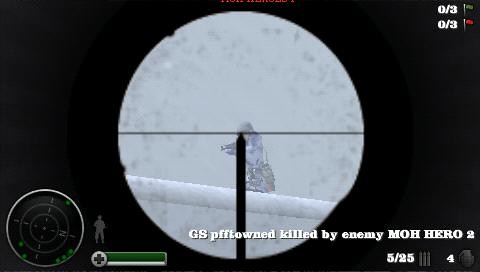The image displays a still from a military-themed video game, characterized by a predominantly black background. Central to the scene is the view through a sniper rifle scope, marked by a white circle with crosshair lines intersecting horizontally and vertically. The scope is focused on a distant, faded soldier dressed in military gear, possibly World War II, who appears to be standing on a rooftop. He's aiming his rifle toward the left side of the screen. To the left of the scope, there's a compass with a black center, light gray directional markings, and green indicator dots. Next to it is a health bar, half-green and half-gray. An interface at the bottom shows the text: "G.S.P.F.F.L.O.W.N.E.D., KILLED BY ENEMY, M.O.H. H.K.R.O.2." Alongside this, there are several gameplay indicators: "5/25", three vertical gray lines, "4", and a small gray circle in the bottom-right corner. The right side of the screen displays "0/3" with a green flag and "0/3" with a red flag, adding context to the game's scoring or objective system. The entire background of the image remains stark black, further drawing focus to the action within the scope.